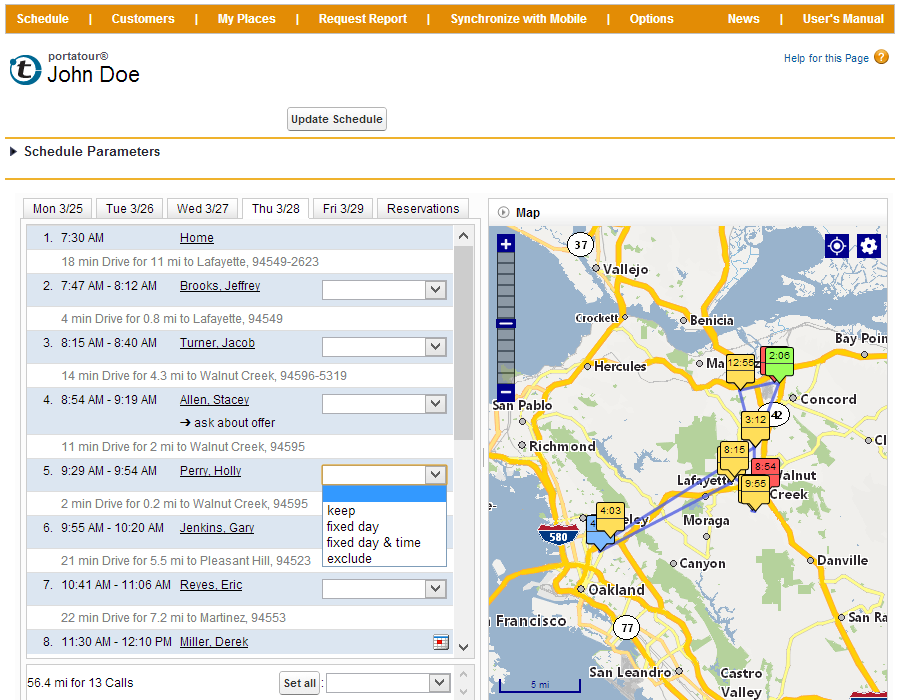**Detailed Descriptive Caption:**

The image is a detailed screenshot of a scheduling application interface with a clean white background. At the top, there is a white header bar featuring an orange strip along its top edge. This header includes several drop-down sections labeled from left to right as follows: "Schedule," "Customers," "My Places," "Request Report," "Synchronize with Mobile," "Options," "News," and "User's Manual." 

Beneath this header, on the left side, is a logo represented by a "T" encircled within a circle, labeled "Port-A-Tour John Doe." Positioned centrally on this banner is an "Update Schedule" button, and towards the right, there is a "Help for this page" link with a question mark icon.

Below the banner, the screen is divided into two main sections. On the left-hand side, there is a tabbed chart or calendar detailing the schedule for the week. The tabs are labeled from left to right as follows: "Monday 325," "Tuesday 326," "Wednesday 327," "Thursday 328" (which is highlighted), "Friday 329," and "Reservations." This section includes a vertical scroll bar on its right edge and lists eight entries, each showing specific times and corresponding names.

On the right-hand side of the image, there is a detailed map marked with various colored icons (red, green, and yellow) indicating different directions. The map itself is rendered in multiple colors including yellow, blue, red, and green, providing a vibrant and clear visual aid for navigation and location identification.